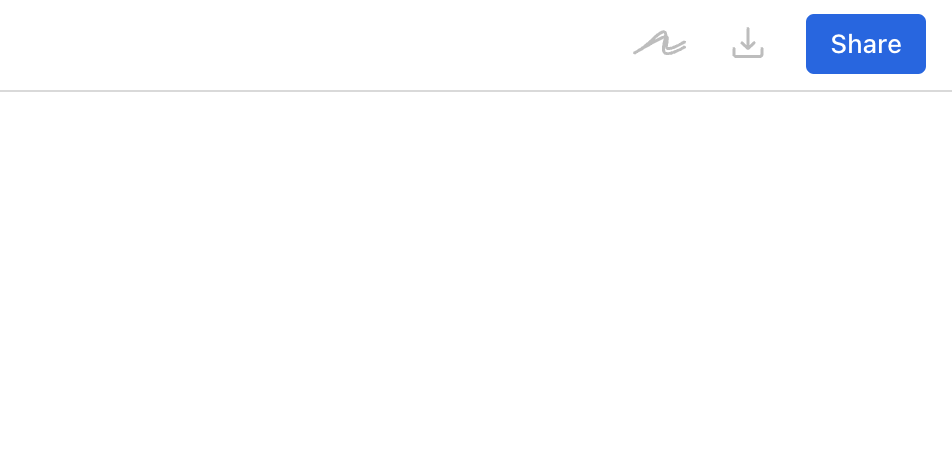In this screenshot, we are presented with an exceptionally minimalistic and unadorned interface. The background is entirely solid white, devoid of any variations or shadows. In the upper-right corner, we see a light gray double-line icon that resembles a wave on water, conveying a simplistic design element. Adjacent to the wave icon, there is a dropdown arrow, hinting at additional options or actions. 

Further to the right, a prominent blue rectangular action button with white centered text reads "Share," inviting user interaction. Directly beneath this suite of icons and the action button, a slender horizontal line in light gray extends from the left to the right edges of the screen, demarcating the header from the lower portion of the page. Below this dividing line, the remainder of the screen continues as a solid, uninterrupted white space, entirely free of text, images, or any other elements. The overall aesthetic is stark and understated, delivering a clean, distraction-free impression.